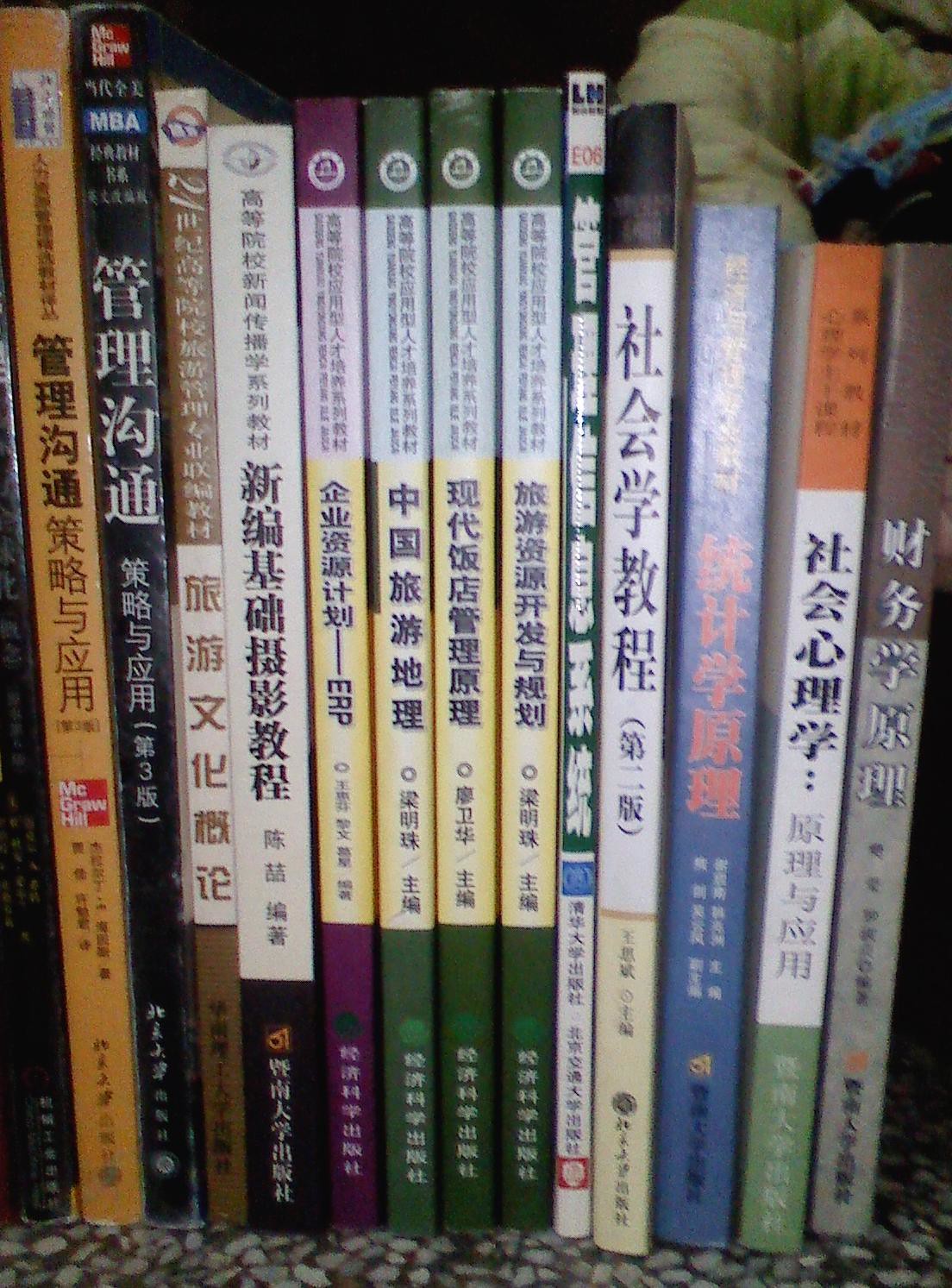This close-up photograph captures a neatly arranged row of thirteen vertically standing books, each about half an inch thick. The books, varying in colors—green, blue, orange, brown, gray, yellow, and black—display Asian characters on their spines, predominantly in either Chinese or Japanese. Among them, a noticeable set of three or four books shares a uniform green color, suggesting they belong to a series or different parts of the same story. The books rest on a distinctive black shelf with white spots, which might be a patterned surface or granite with a speckled design. Behind the books, a light green lily flower adds a subtle touch of elegance to the scene, and the image is illuminated by light reflecting off the books, indicating it was shot indoors.